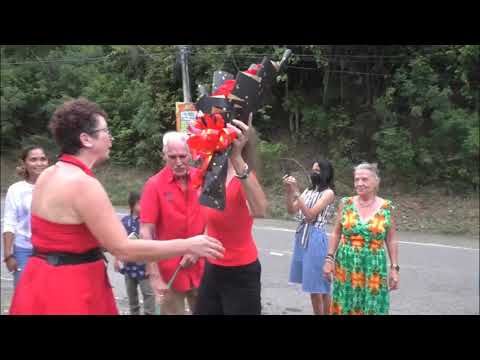The image captures a lively scene of seven people gathered by the side of a road, which stretches across the foreground with its clean white stripes and an absence of traffic. The road is bordered by a forested hillside, contributing to the serene backdrop. Central in the image is a woman wearing a red dress with a black belt, brown hair, and glasses, extending her arms towards another woman in a red shirt and black pants who is handing her a peculiar black object adorned with gold triangles and red ribbons, resembling a piñata or a paper bouquet. 

Behind them, a man in a red short-sleeved button-down shirt and khaki pants looks on, while nearby, a woman in an orange and green floral sundress is watching with a smile. On the far right, a woman with long black hair, wearing a black medical mask and a blue skirt with a black and white sleeveless top, appears to be capturing the moment with a camera. Further back, another woman is visible, dressed in a red and purple sweater with lavender pants, also smiling at the ongoing interaction. A young boy in a blue shirt and tan pants stands by a street sign, and to the far left, partially hidden, there is a young woman with brown hair tied back, wearing a white shirt and blue pants. The scene suggests a shared moment of curiosity and interaction among the group in a picturesque outdoor setting.